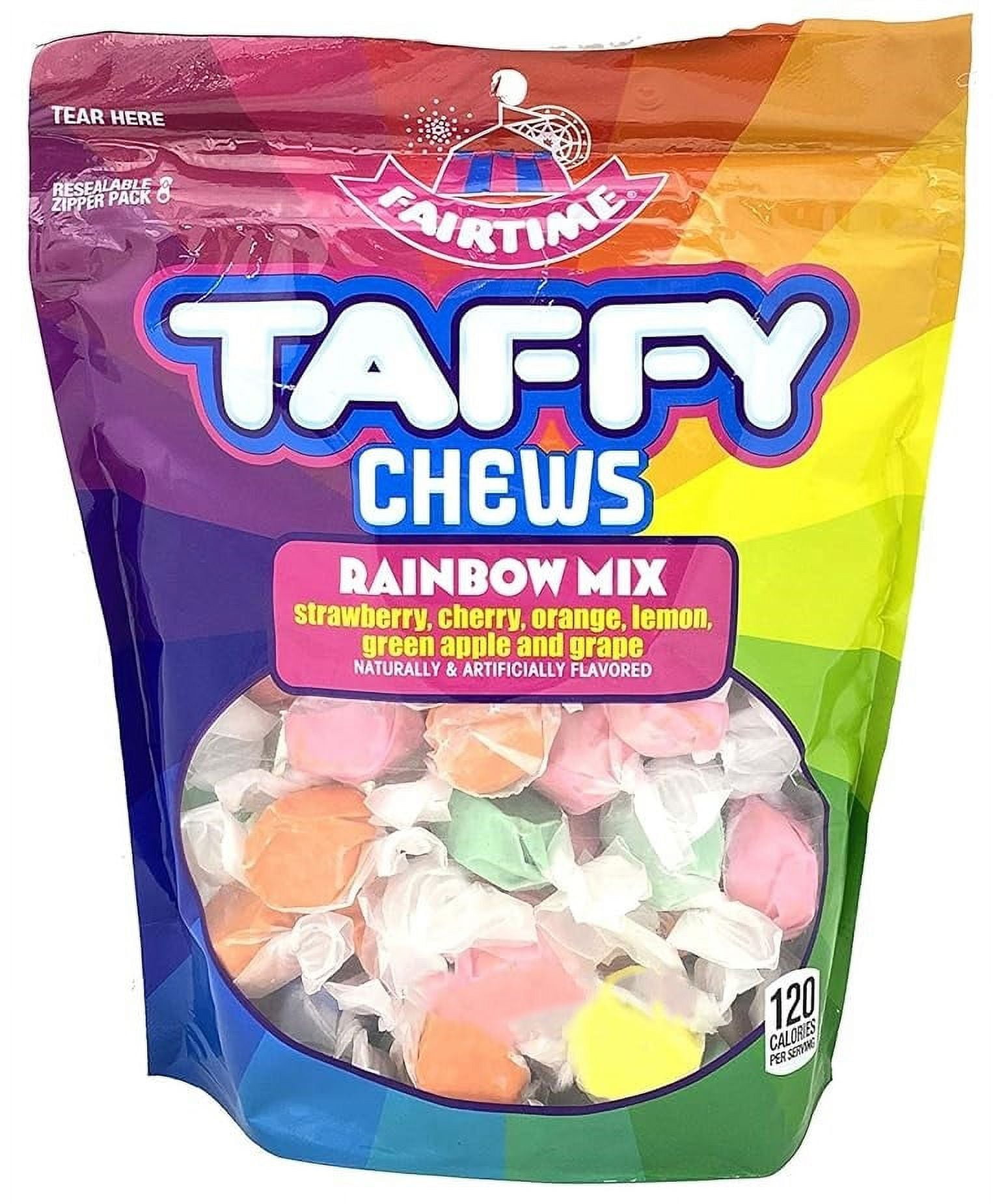This image features a colorful, plastic bag of taffy candies titled "Fair Time Taffy Chews." The bag is adorned with a vibrant rainbow gradient, beginning with hues of orange, yellow, and green on the right-hand side, transitioning through blue, purple, and red as you move to the left-hand side in a clockwise pattern. 

The top of the bag showcases a small, green logo above the product name written in large, white, marshmallow-like letters with a black border. Below the main label, the words "Taffy Chews" are prominently displayed. A pink text box with white lettering labels the candy as "Rainbow Mix." The assorted flavors listed on the package, displayed in yellow text, include strawberry, cherry, orange, lemon, green apple, and grape. 

Additionally, the bag features an elliptical clear section in the center, allowing a view of the colorful, wax-wrapped candies inside. The packaging also notes the flavors as both "naturally and artificially flavored," and indicates that there are 120 calories per serving. The bag is set against a plain white background, emphasizing the bright, eye-catching design and contents.